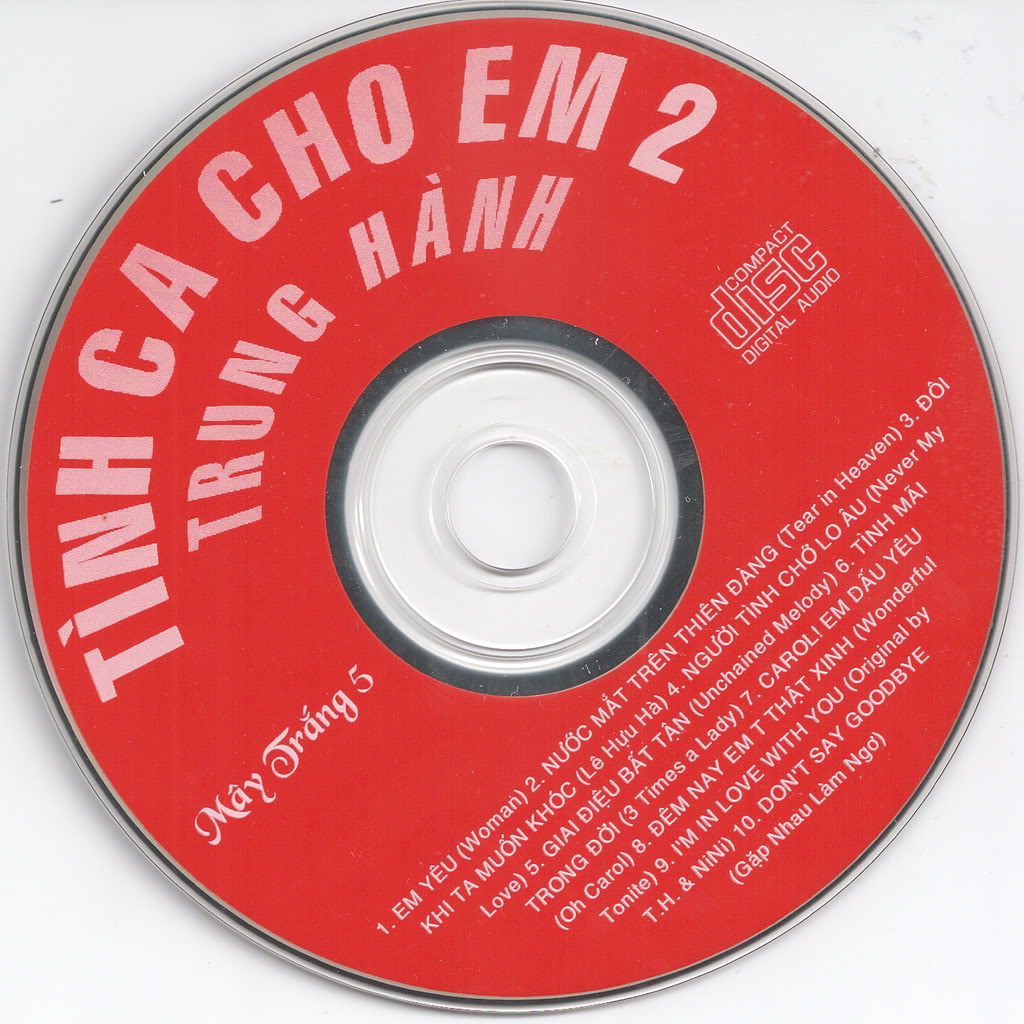This square image features a vibrant red compact disc showcased against a light gray background, which subtly transitions to white at the bottom corners. The CD takes center stage, shadowed slightly on its lower left side. The disc itself has a clear central hole surrounded by a black border, radiating into the red surface dominated by white text. Diagonal from the bottom left to the top right, the central text reads "TINH CA CHO EM 2 TRUNG HANH". On the left side of the disc, "Mae Trang 5" is inscribed, while the right side is marked with "Compact Disc Digital Audio". At the bottom, there's a list of ten song titles in Vietnamese, followed by their English translations. The tracklist includes titles such as "MU" (Woman), "Tear in Heaven", "Foreign", "Never My Love", "Unchained Melody", "Something I can't pronounce", "Three Times Lady", "Oh Carol", "Wonderful Tonight", "I'm In Love With You", and "Don't Say Goodbye". This detailed presentation captures both the visual and textual elements of the CD, blending information from multiple descriptions into a cohesive narrative.